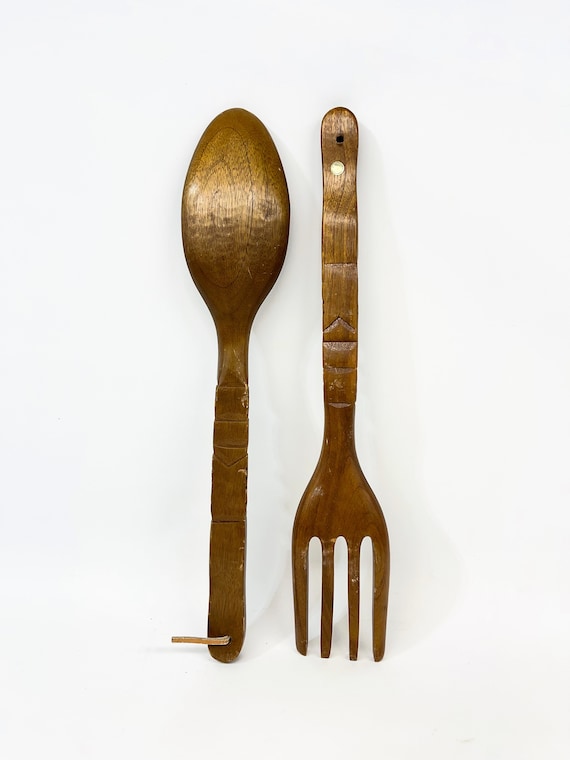This photograph features two intricately designed wooden utensils positioned with their handles adjacent and parallel to each other. On the left, a wooden spoon lies face down with its smooth, rounded back displayed prominently, adorned by a small strap looped through a hole at the end of its handle. On the right, a wooden fork is arranged inversely with its four tines facing downward. Both utensils feature a harmonious golden brown hue with a polished sheen, highlighting their craftsmanship. The handles of both the spoon and fork are carved with decorative engravings, including lines and a distinct triangular pattern, suggesting an antiquated or artisanal quality. The background of the image remains indistinct, possibly suggesting a tabletop view from above, giving prominence to the historical or handcrafted essence of the utensils.